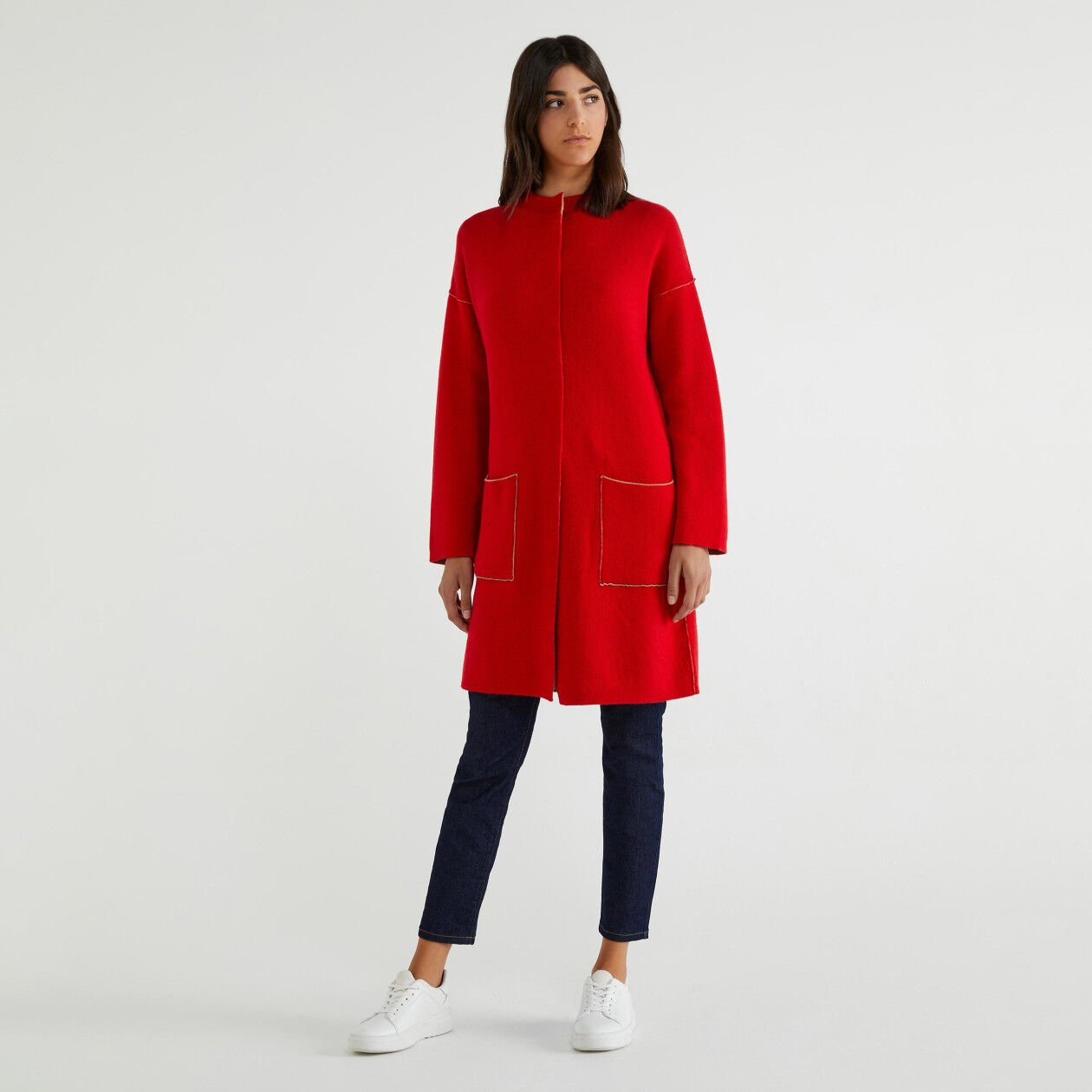In this striking color photograph, a woman sits gracefully in the exact center of the image, against a seamless and minimalist, light gray background that extends to the floor, enveloping her in a serene, almost ethereal ambiance. She gazes solemnly off to her left, the right side of the photograph, giving the impression of introspective contemplation. Her long, straight, dark brown hair cascades past her shoulders, contrasting with her distinctive outfit. She dons an unusual, long red coat with over-large pockets positioned low at the front; the coat stands out due to its lack of visible zippers, buttons, or connectors, yet it remains closed. Paired with the coat are snug blue capri jeans, revealing her bare ankles above her white tennis shoes. The image exudes a high-fashion, editorial vibe, reminiscent of a magazine spread, emphasized by the focused isolation of the model and the expansive blank space surrounding her.